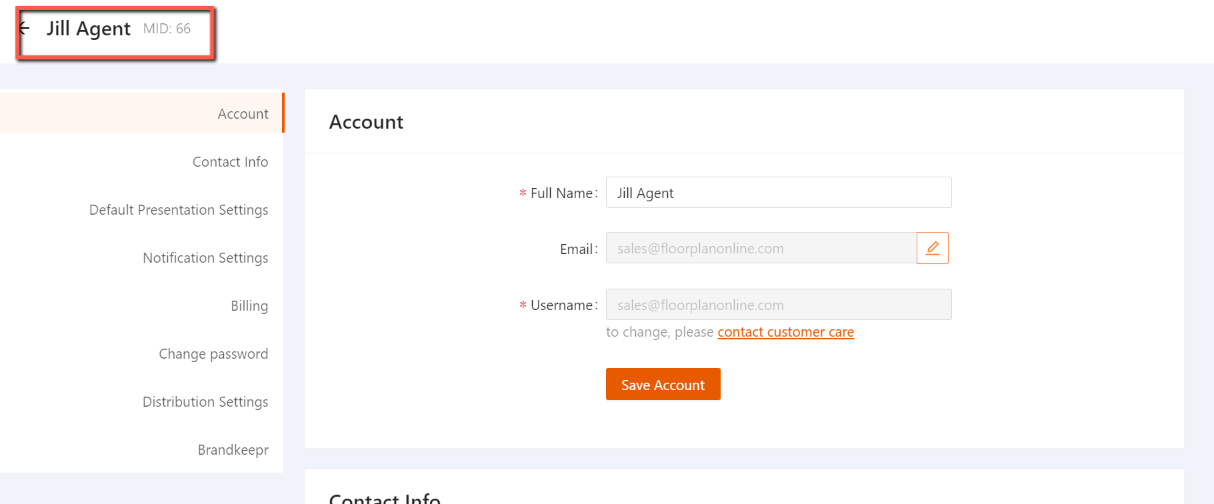The image is a detailed screen capture of an online account settings page.

At the top of the screen, within a white banner, there's a black back arrow followed by the text "Jill Agent MID-66" highlighted in a red box. Below this banner, a white menu lists several gray-colored categories, one of which is highlighted in tan. The categories read: Account, Contact Info, Default Presentation Settings, Notification Settings, Billing, Change Password, Distribution Settings, and Brand Keeper. A visible red scroll bar is positioned alongside the menu.

Further down, a large white box contains various text fields and options. The first field, labeled "Full Name" in black text with a red asterisk, displays "Jill Agent." Beneath it, the "Email" field appears within a gray box, featuring an orange pencil icon and the text sales@floorplanonline.com. The next field shows the username as sales@floorplan.com. Instructions to change the username are provided in gray text, indicating to "contact customer care" in orange. An orange and white box at the bottom of the section reads "Save Account."

At the very bottom of the image, the text "Contact Info" appears in black, and the image cuts off shortly after this point. Surrounding the described elements is a faint gray border. The text within the image is clear and easy to read. No further notable elements are present.